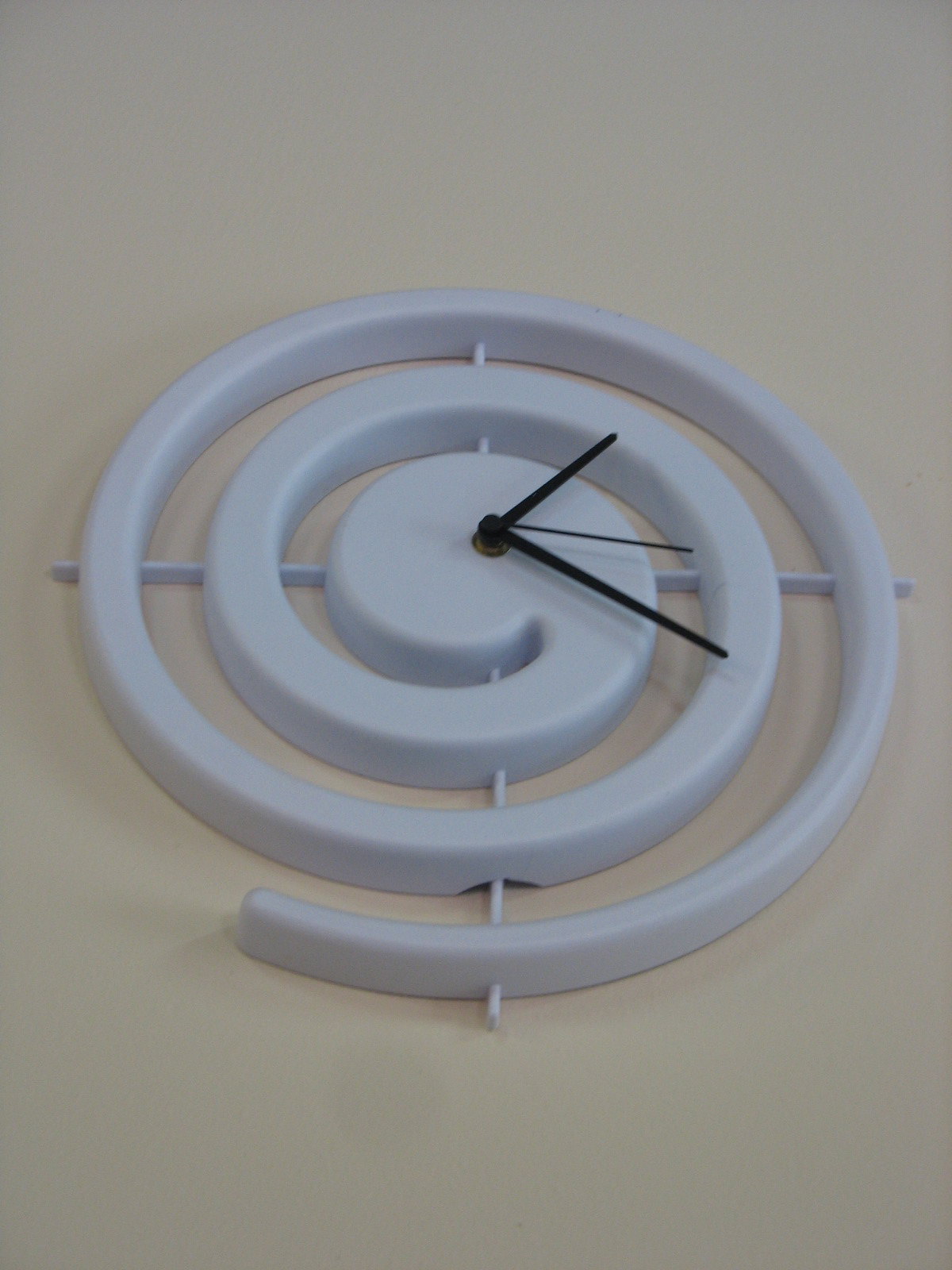The photograph depicts a unique, artistic clock face against a neutral off-white or cream-colored wall, captured from a low angle looking up. The clock, which appears to be made of white plastic, features a striking spiral design. This spiral begins near the seven o'clock position and gracefully coils inward through multiple loops to terminate at the center. The central part of the swirl, thicker and more defined, hosts the black hour, minute, and second hands, indicating a time of approximately twenty minutes past one. Notably, the clock lacks any numerical indicators or markings, requiring familiarity with traditional clock positions to read the time. In the background, thin white bars form a subtle plus sign, providing structural support to the overall design.